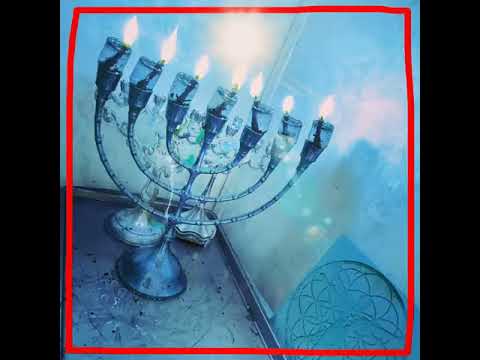This image features an artistically rendered menorah, characterized by seven lit candles arranged in a series. The menorah, predominantly in various shades of blue, stands out against a light blue background and is set at an angle within the composition. It has glassy blue candle holders, each with a glowing flame, reflecting onto the adjacent wall. Surrounding the image is a hand-drawn, somewhat irregular red border, giving it a unique, possibly AI-generated or painted appearance. Behind the primary menorah, there appears to be a smaller silver menorah and other candle holders, though these are somewhat indistinct. The menorah rests on a surface that resembles a tray, and the entire scene is illuminated by the candles, casting shadows and adding depth. In the bottom right corner of the image, there's a circular design, adding an additional decorative element to the scene. The overall presentation resembles an album cover or a digitally crafted artwork.